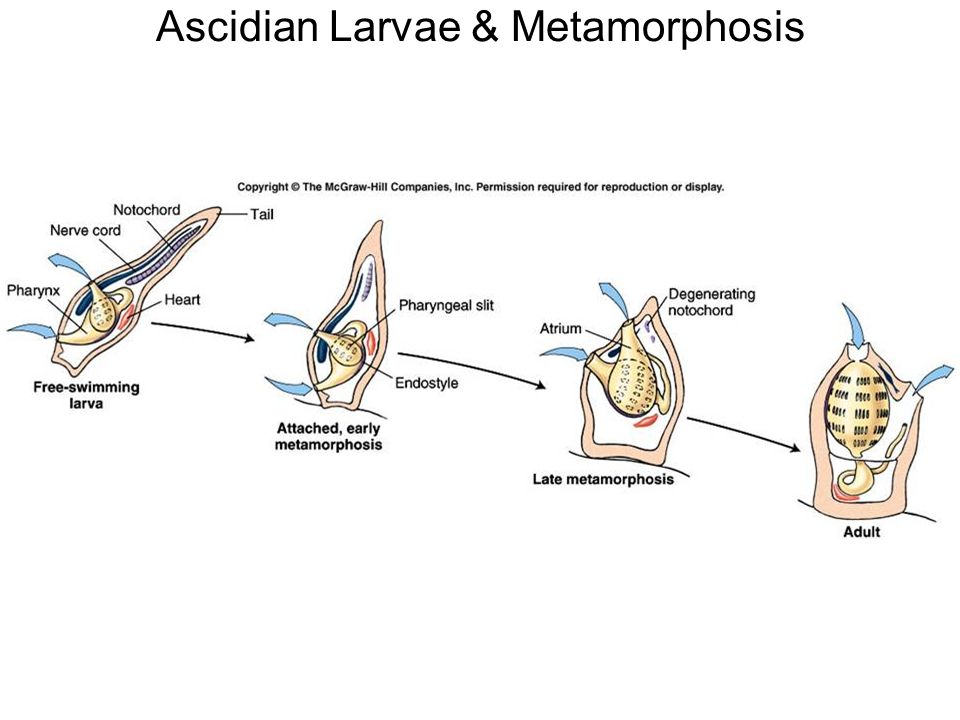The scientific diagram illustrates the stages of ascidian larva metamorphosis, transitioning from a free-swimming larva to an adult. The sequence is detailed as follows: the free-swimming larva, characterized by a tail, nerve cord, pharynx, and heart, is depicted in a yellowish-beige color and is accompanied by labeled annotations. As the larva progresses to early metamorphosis, significant transformations occur, including the movement of the heart. This stage includes labels for the endostyle and pharyngeal slit. In the late metamorphosis stage, features such as a degenerating notochord and the formation of an atrium are highlighted. Finally, in the adult stage, the heart relocates to the bottom while the pharyngeal slit forms the primary structure of the main body. Surrounding each image are arrows that illustrate the developmental changes, emphasizing the increasing roundness and plumpness of the organism at each stage. The diagram also includes a copyright notice from McGraw-Hill Companies, indicating permission is required for reproduction or display.